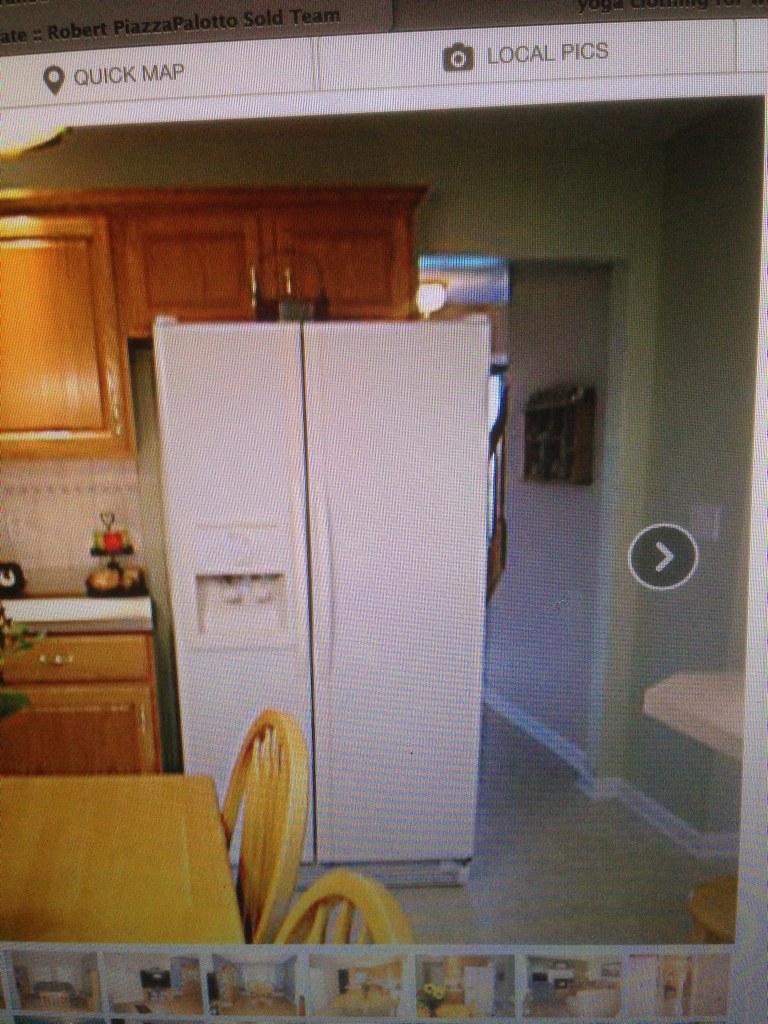The grainy vertical image, seemingly a screenshot of a real estate website like Zillow, captures the interior of a kitchen in a house listing. At the top left corner of the browser window, a gray tab displays the text "Robert Piazza, Pelota, sold team," with navigation buttons labeled "QuipMap" and "Local Picks" featuring a camera and map emoji respectively. Dominating the center is a detailed view of a kitchen featuring a side-by-side white refrigerator with an ice maker and water dispenser. The backdrop includes light green walls and medium brown wooden cabinets topped with a cabinet above the fridge. Below, a counter with a fruit stand, a drawer, and a door sits adjacent to a light wooden table accompanied by similarly light wooden chairs with rounded backs. The kitchen’s beige flooring is trimmed with white. At the bottom of the screen, there are thumbnails of six additional rooms, underscoring that this is a still from a digital property listing.